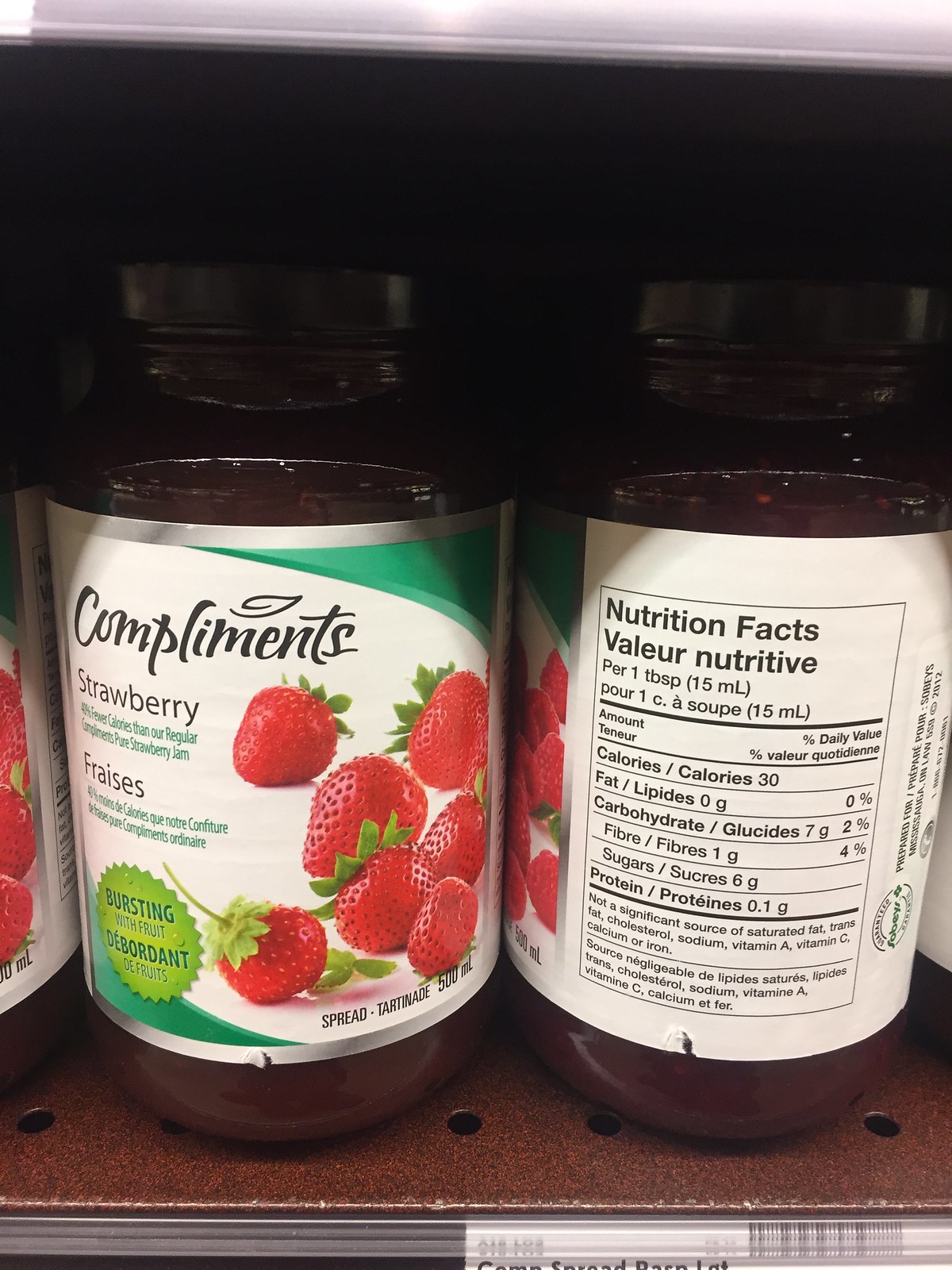The image depicts two glass bottles on a brown shelf. The shelf has noticeable holes along its bottom edge and a glittery brown finish. Both bottles are identical, but their orientations differ. 

The bottle on the right is facing the back, showcasing a white sticker with detailed Nutrition Facts in tabular form. The container holds a maroon-colored substance.

The bottle on the left is displayed from the front. Its white label features a combination of black, green, and red colors, including an illustration of red strawberries with green leaves. At the top, the word "Compliments" is printed in black, followed by "Strawberry" in green and "45% fewer calories than our regular." The label further reads "Compliments Pure Strawberry Jam," with a phrase about a 40% reduction in another language. Additional text at the bottom of the label indicates "Best thing with fruit" in green, along with "Spread, 500ml" in the bottom right corner.